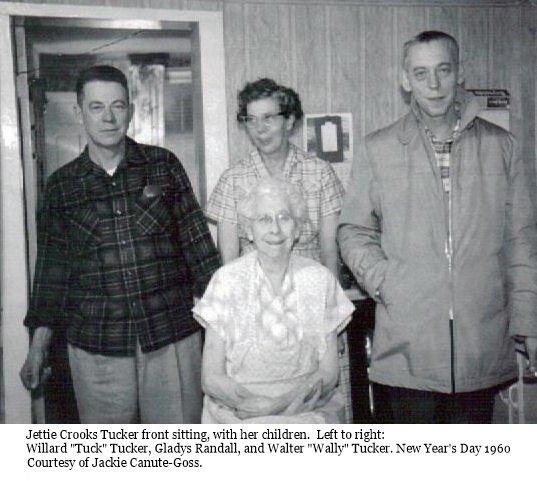This detailed black and white photograph depicts a family gathering inside a room, likely a kitchen, captured on New Year's Day, 1960. The image shows four people: an older woman seated in the front center and her three children standing behind her. From left to right, we see a man identified as Willard Tuck Tucker, a woman with glasses named Gladys Rendell standing in the middle, and another man named Walter Wally Tucker on the right. Behind the family, the wall and a door of the room are visible. Below the photograph, text reads: "Jetty Crooks Tucker front sitting with her children left to right: Willard Tuck Tucker, Gladys Rendell, and Walter Wally Tucker. New Year's Day, 1960. Courtesy of Jackie Knut Gose." The grayscale tones highlight the period style and the intimate family moment captured decades ago.